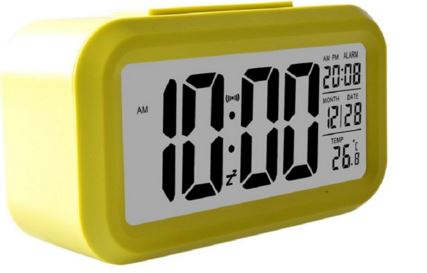This photograph showcases a yellow, oblong-shaped digital alarm clock with a rectangular overall body featuring rounded edges. The clock is angled slightly to the right, with a bright light illuminating the left side. Its white face displays bold black print, showing the current time as 10 AM, with an "AM" indicator highlighted on the left. Additional details on the display include the date "2008-12-28," a temperature reading of "26.8°C," and various symbols such as a sound icon and a "ZZZ" symbol indicating sleep mode. The yellow casing is distinctive, with a bar on top, likely for snooze functions. The white background further accentuates the clock's vibrant appearance.